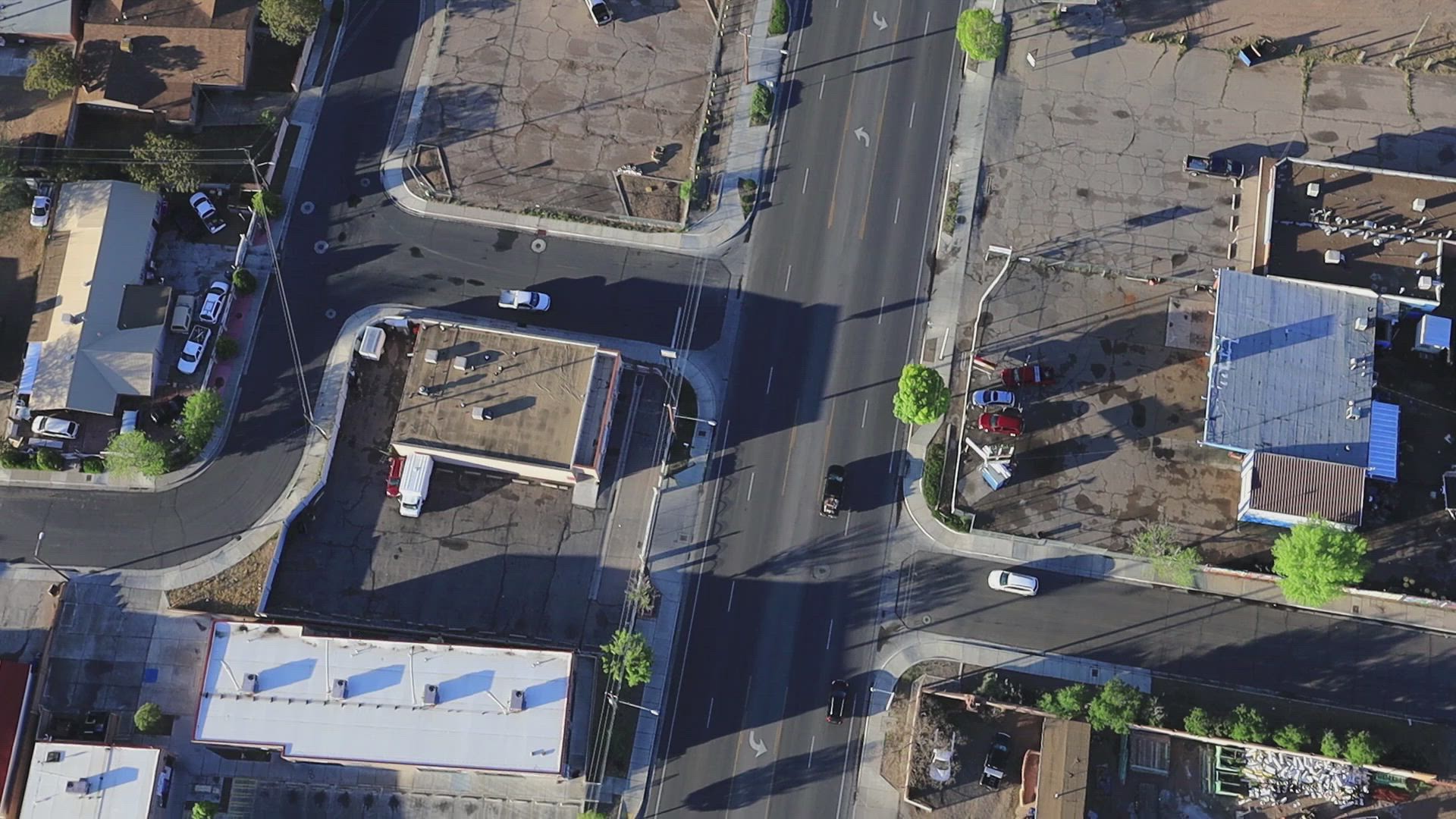An aerial photograph captures a busy urban T-intersection from a considerable height, likely from a helicopter or drone. The main thoroughfare, running vertically, features two lanes in each direction with a central turn lane. A secondary road enters from the lower right, with two lanes, typical of a side street joining a main road. 

Lining both the main and side roads are several trees, with a higher concentration along the side road. On the left side of the image, flat-roofed buildings dominate the scene, appearing to be commercial enterprises rather than residential homes. Prominently, a warehouse-like building, situated in the middle left, has air handling units on its roof and a truck positioned at a loading dock.

Another road enters from the bottom left, curving upward to join the main thoroughfare. Adjacent to this road's curve, a secondary road branches off towards the main thoroughfare, passing by the warehouse.

In the top-middle of the photograph lies an extensive, cracked asphalt parking lot, surrounded by a potential fence with planted borders and sidewalks. The lot seems largely vacant of buildings within the frame.

On the far left, more commercial buildings are evident with numerous cars parked in front, suggesting a bustling warehouse district.

On the right side, another vast, cracked asphalt parking lot contains a few scattered cars, adjacent to a complex of flat-roofed buildings. Near the bottom right, smaller buildings, possibly houses, are separated from the sidewalk by a row of trees planted along a fence.

Vehicle activity is minimal, with two dark-colored cars on the main thoroughfare and a single white vehicle on the side road nearing the intersection. Another white car approaches the intersection from the opposite side of the thoroughfare. The sun casts long shadows from the trees, vehicles, and rooftop air handlers, indicating a bright, sunny day.